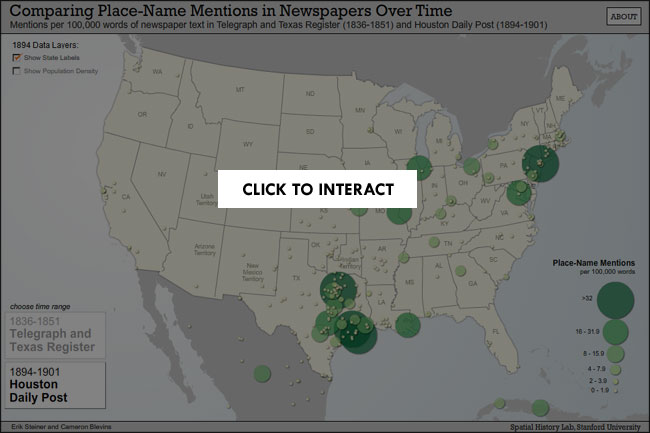The screenshot depicts a section of a website or a web-based application, designed in the shape of a computer screen, without a visible browser URL. Dominating the screen is a detailed map of the United States, positioned centrally. This map features a white background with gray lines marking each state's borders, and state initials neatly placed within their respective boundaries. 

Surrounding the United States map, Canada to the north and Mexico to the south are visible, though they appear as blurred, indistinct shadows, providing context without drawing attention from the main focus.

Scattered across the U.S. map are numerous green circles of varying sizes. These circles indicate place name mentions per 100,000 words in historical newspapers. The legend, located to the right, clarifies that smaller, lighter circles represent fewer mentions, while larger, darker circles signify higher mentions. The largest circles indicate more than 32 mentions per 100,000 words.

At the top of the screenshot, a title reads "Comparing place name mentions in newspapers over time." Specifically, the data spans mentions per 100,000 words of newspaper text from the "Telegraph and Texas Register" (1836-1851) and the "Houston Daily Post" (1894-1901). This detail provides a historical context, highlighting how frequently various U.S. locations were mentioned in these particular publications during the specified years.